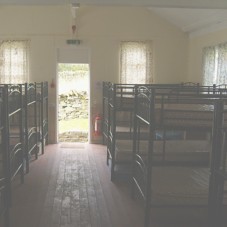This small square photograph captures the interior of a bunkhouse, vividly showcasing its modest but functional setup. The room features two rows of black-framed bunk beds with white mattresses, three on the left side and three on the right. The floor, covered in wooden panels of a reddish-brown hue, guides the eye towards an open door at the end of the aisle, allowing sunlight to pour in. Flanking the door are two windows, each adorned with white sheer curtains, and a third window is positioned on the far right wall, also with sheer curtains. The walls are light, possibly white, adding to the brightness of the room. Above the door, there appears to be a white object, possibly a light fixture, though it is not illuminated. A faded fire extinguisher is mounted on the lower right side of the doorway, adding a touch of safety functionality to the space. The scene is one of utilitarian simplicity, with an emphasis on practicality and order.